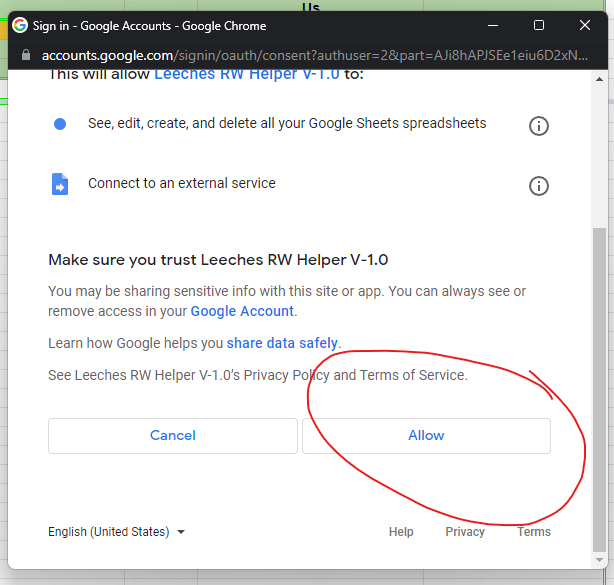The image is a screenshot of a website page for Google account sign-in, featuring various elements and instructions. At the top of the page, the Google logo is prominently displayed in its signature red, yellow, green, and blue colors. To the right of the logo, options for "Sign in," "Google Accounts," and "Google Chrome" are listed.

Next to these options are three symbols typically found in a browser window: a dash to minimize the window, a square to resize it, and an "X" to close it. Below these symbols, a padlock icon indicates a secure connection. The URL displayed is "accounts.google.com" in white letters, followed by a long, grayed-out extension.

The main content of the webpage describes permissions for an application named "Leech's RW helper." It states: "This will allow Leech's RW helper…" but the rest of the sentence is cut off. Below this partial sentence, a blue dot is visible, followed by the text: "See, edit, create, and delete all your Google Sheets spreadsheets." Additionally, there's a circle with an "i" inside it, possibly for more information.

Further down, an icon resembling a blue sheet of paper with an arrow is labeled "Connect to an external service." The heading underneath reads: "Make sure you trust Leech's RW helper V-1.0," accompanied by a warning about sharing sensitive information. The text explains that users can always see or remove access in their Google account, with clickable links for "Learn how Google helps you share data safely" and "Google account and share data safely," both highlighted in blue.

The following line offers links to the privacy policy and terms of service for "Leech's RW helper V-1.0." At the bottom, two buttons are available: "Cancel" and "Allow." The "Allow" button is notably circled in red with an editing pen, indicating user attention or action. Lastly, the footer shows standard website links: "English (United States)," "Help," "Privacy," and "Terms."